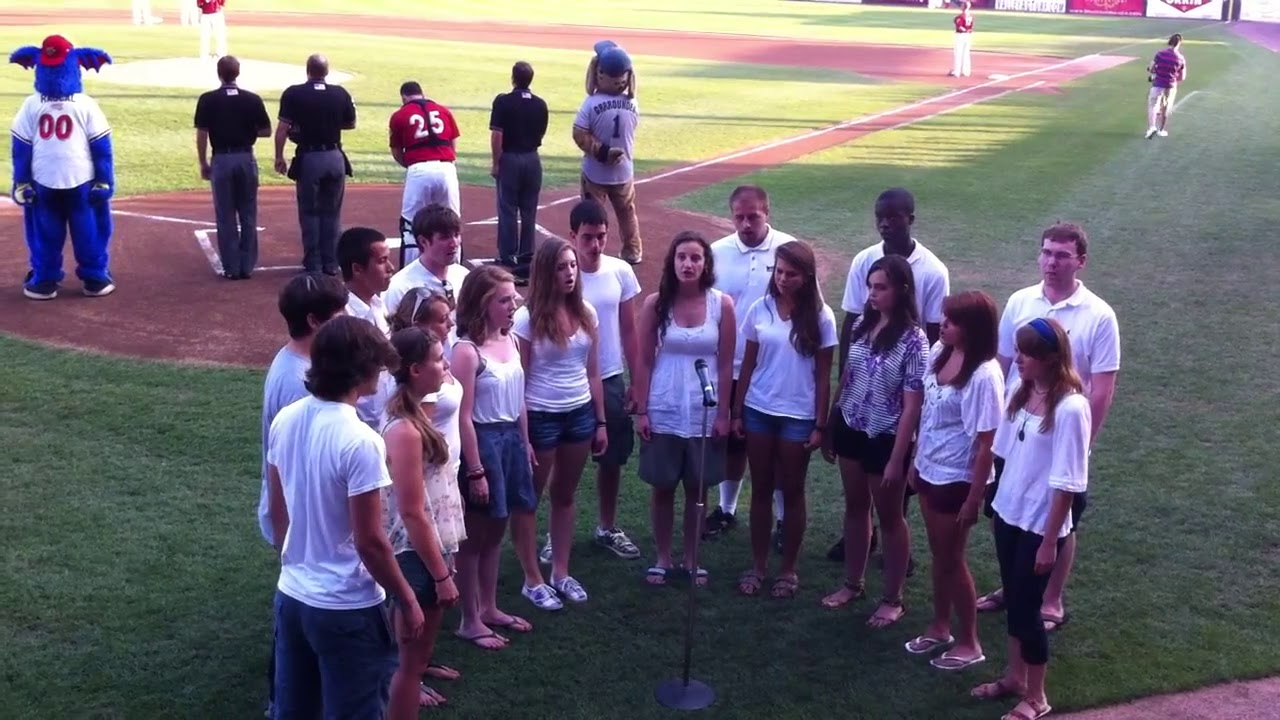In this vibrant daytime photograph of a baseball field, a choir of young men and women is standing in a semicircle behind home plate, singing presumably the National Anthem. They are dressed primarily in white shirts or light clothing and jean shorts, facing the camera with a microphone in the center. The home plate area, shaded from the sun, forms the backdrop where three umpires and a catcher in a red jersey with the number 25 can be seen with their backs turned. Two team mascots add a playful touch—the first, a blue character with bat-like ears and a red backwards baseball cap, and the second, possibly a dog with floppy ears. The sun illuminates the pitcher's mound further up the field, casting a serene light on the otherwise shaded participants. The lush green grass around home plate and the brown dirt of the field create a rich, contrasting surface for this pre-game moment.